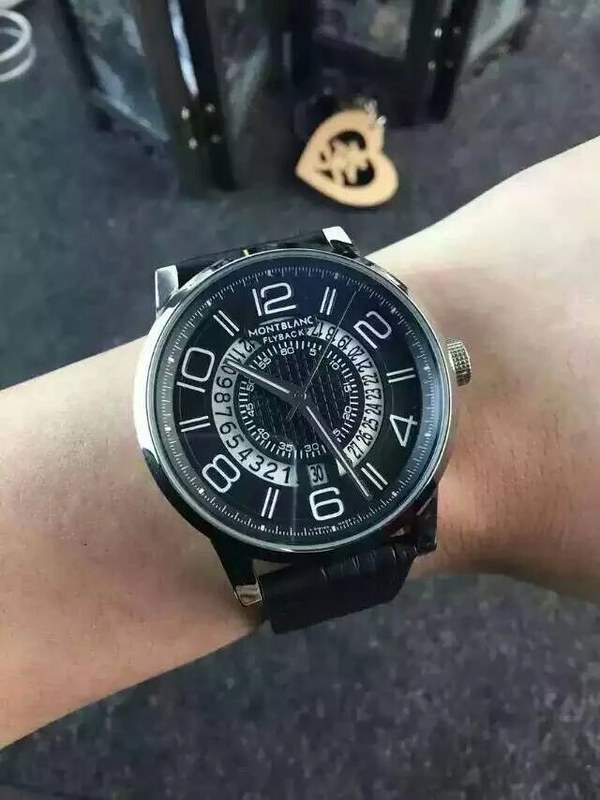A close-up image captures a Montblanc flyback watch elegantly positioned on someone's left wrist. The sophisticated timepiece features a black leather band and a silver case, exuding a sense of refined luxury. Its intricate bezel is composed of alternating black and white rings, each serving distinct time-telling functions. The innermost ring displays measurements in intervals of 10, 11, 15, and 20, while the middle ring denotes individual minutes from 1 to 3. The outermost ring indicates the hours at 12, 2, 4, 6, 8, and 10, marked by double slashes at the odd hours for 1, 3, 5, 7, 9, and 11. The sizable face of the watch dominates the composition, with detailed watch hands and sub-dials adding to its complexity. Though slightly blurred, the background reveals what appears to be a piece of jewelry or a Japanese-style screen, adding an additional layer of sophistication and context to the setting. The primary focus remains on the watch, highlighting its design and craftsmanship against the subtle backdrop.